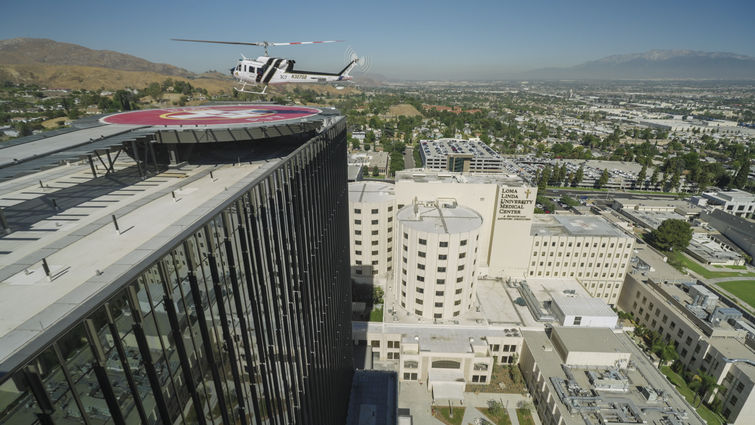This is a high-altitude, horizontal color photograph of Loma Linda University Medical Center in Southern California, likely taken from another tall building or by a drone. Dominating the left-hand side is a modern, glass-paneled building with vertical black structures and a flat, white roof featuring a bright red, circular helipad. A white helicopter with black stripes is on the verge of landing on the helipad, indicating the facility's use for critical patient transport. Below and to the center, we see the prominent white buildings of the medical center, marked with the Loma Linda University Medical Center signage, and depicted with cylindrical structures and a cross. The surrounding cityscape, with its mix of shorter buildings, extends into the background, merging into foothills—dry and brown on the upper left—and a taller mountain on the right. The entire scene is set under a blue sky with a noticeable layer of smog typical of the Southern California atmosphere.